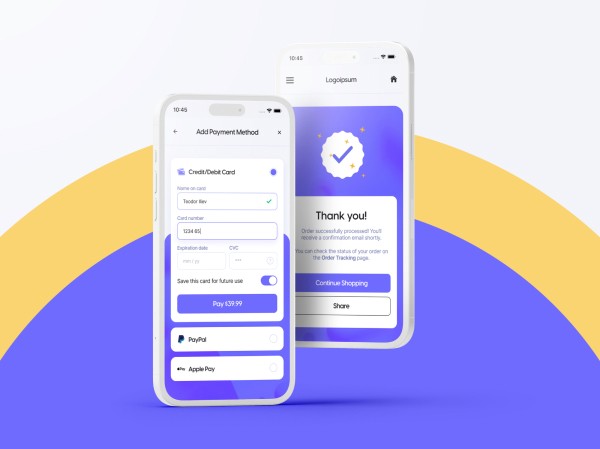This image appears to be a mock-up for an advertisement, possibly intended for a website, promoting a mobile app. The background features a stylized design resembling a rising sun, with a blue half-circle at the bottom, bordered by a golden stripe, and merging into a white upper section. In the foreground, two smartphones are prominently displayed, each showcasing different screens of the app to illustrate its interface and functionalities. The phones are angled for a dynamic visual effect— the one in front is slightly tilted to the right, while the one behind it is slightly tilted to the left. The app's color scheme echoes the blue from the background, creating a cohesive visual theme.